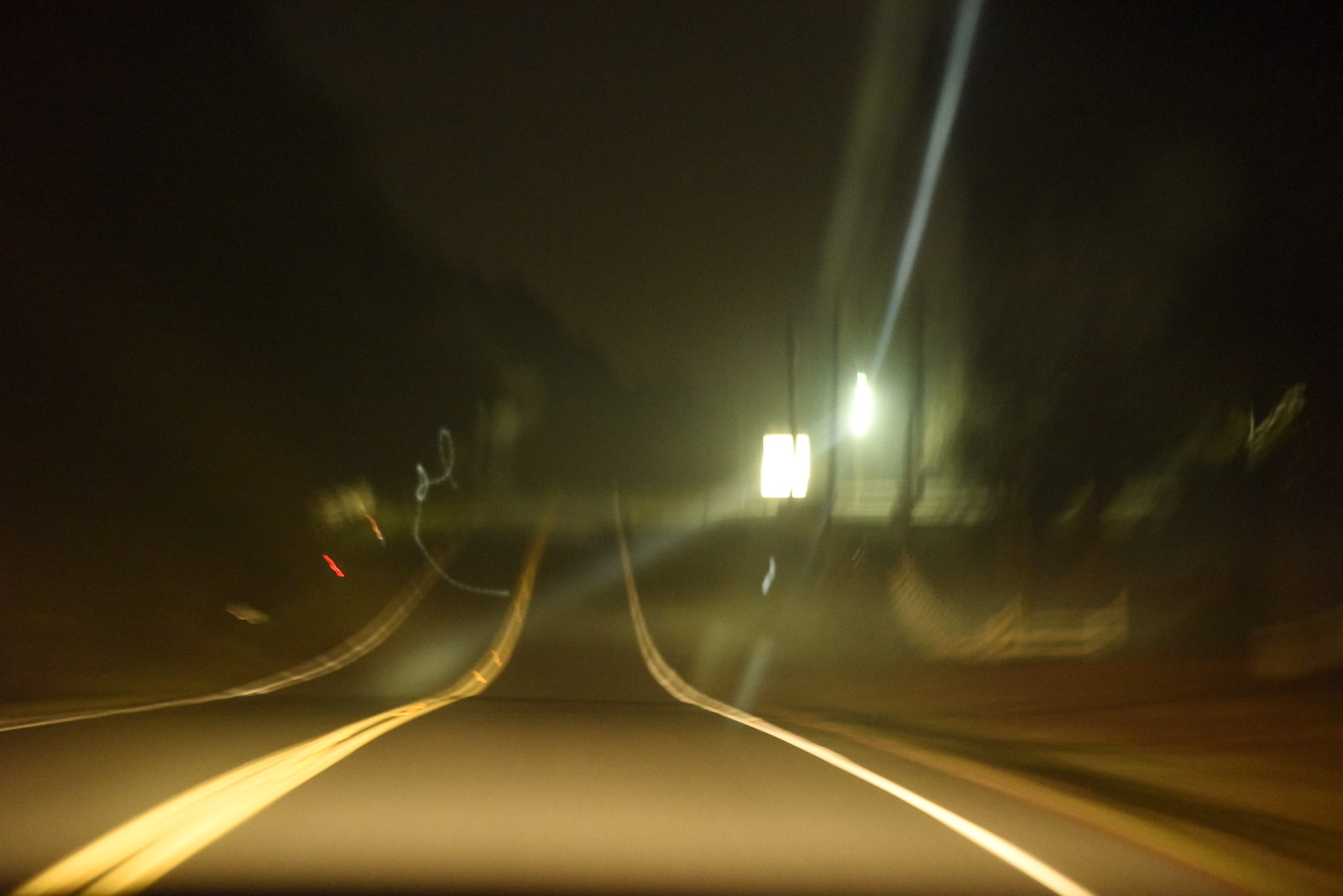A blurred, AI-generated image captures a curving road descending gently before ascending slightly, set against a dark evening sky. Street lights, whose irregular shapes suggest both motion blur and possible computer-generated errors, dot the scene. The road, likely a two-way street, is flanked by blurred trees on both sides. In the background, vague and indistinct structures are visible behind the trees on the left. Overall, the image exudes an eerie, dreamlike quality due to the pervasive blurriness and the dim, twilight atmosphere.